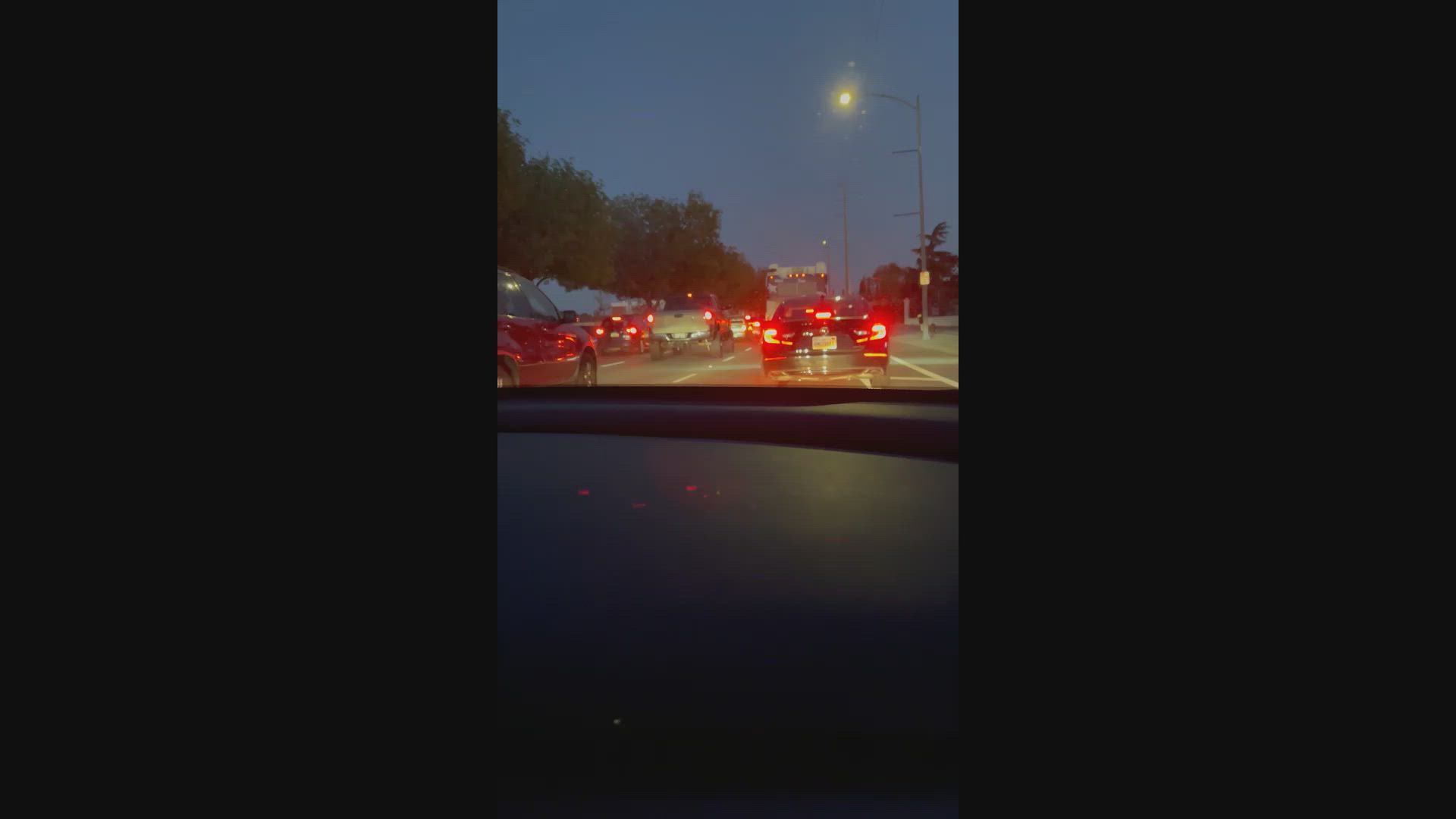A twilight photograph captures the bustle of evening traffic from the perspective of a vehicle's dashboard. The gray dashboard, detailed with subtle textures, occupies the lower half of the image, grounding the viewer in the scene. Above, a three-lane street is crowded with vehicles, their brake lights glowing a vibrant red, creating a striking contrast against the dimming light. The vehicles are all aligned in the same direction, suggesting a potential traffic jam or a prolonged stop at a red light. Beyond the sea of cars, a dark tree line is faintly visible, adding depth to the scene. Street lights cast a gentle glow, illuminating the area without overpowering the remaining natural light. The sky, draped in a rich, dark blue hue, signifies the transition from day to night, perfectly capturing the essence of twilight.